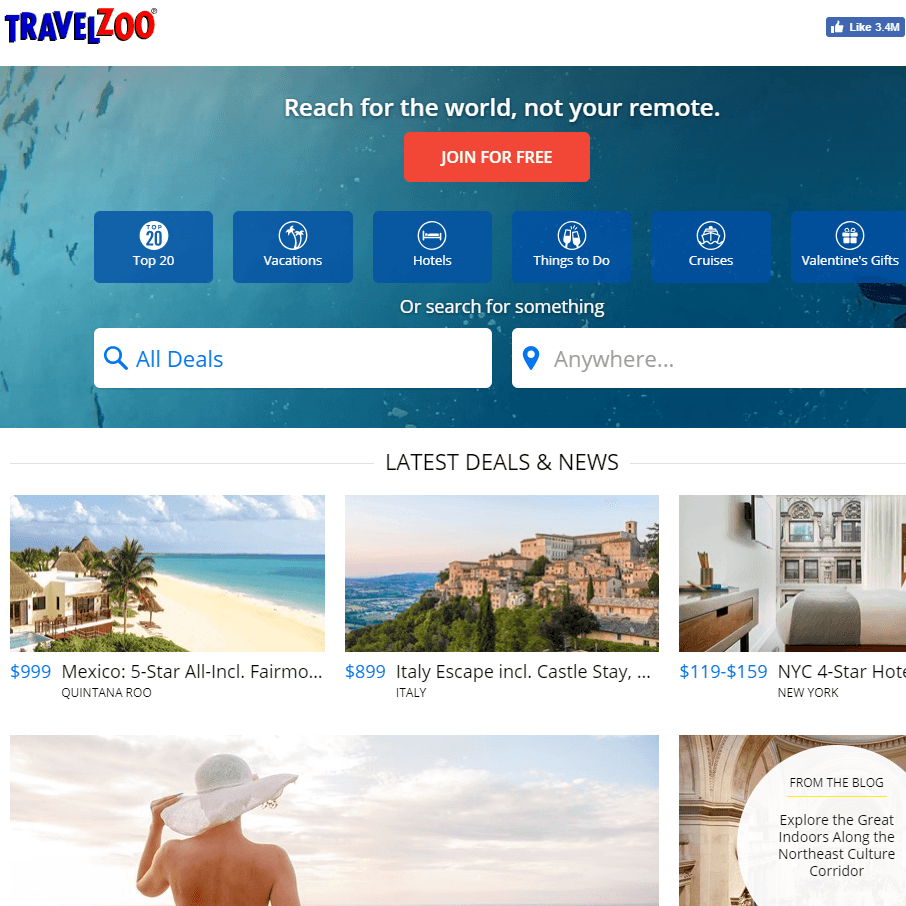Top-left corner features a quirky, uneven logo. The first word, "Travel," is in dark blue font, followed by "Zoo" in red font with a black shadow underneath. There's a registered or trademark symbol at the top-right of the logo.

Below the logo, a banner depicts an underwater scene. In the center of the banner, white text reads, "Reach for the world, not your remote." 

Underneath the banner, an orange, rectangular icon with rounded edges bears the white, capitalized text "JOIN FOR FREE." 

Below this icon, there are several circular boxes with various icons and labels:
- A white circle labeled "Top 20."
- A circle with two palm trees labeled "Vacation."
- A circle with a bed labeled "Hotels."
- A circle with champagne glasses labeled "Things to Do."
- A circle with a boat labeled "Cruises."
- A circle with a present labeled "Valentine's Gifts."

Further down, white text reads, "Or search for something." There are two query options:
- The first query has a blue magnifying glass icon on the left and says "All Deals" in blue writing.
- The second query has a blue map pin with a white circle at the top, labeled "Anywhere..." in light gray lettering. Both queries are editable with text.

Centered below, on a white background, is capitalized text that reads, "LATEST DEALS & NEWS." This text is flanked by long gray lines extending to the left and right.